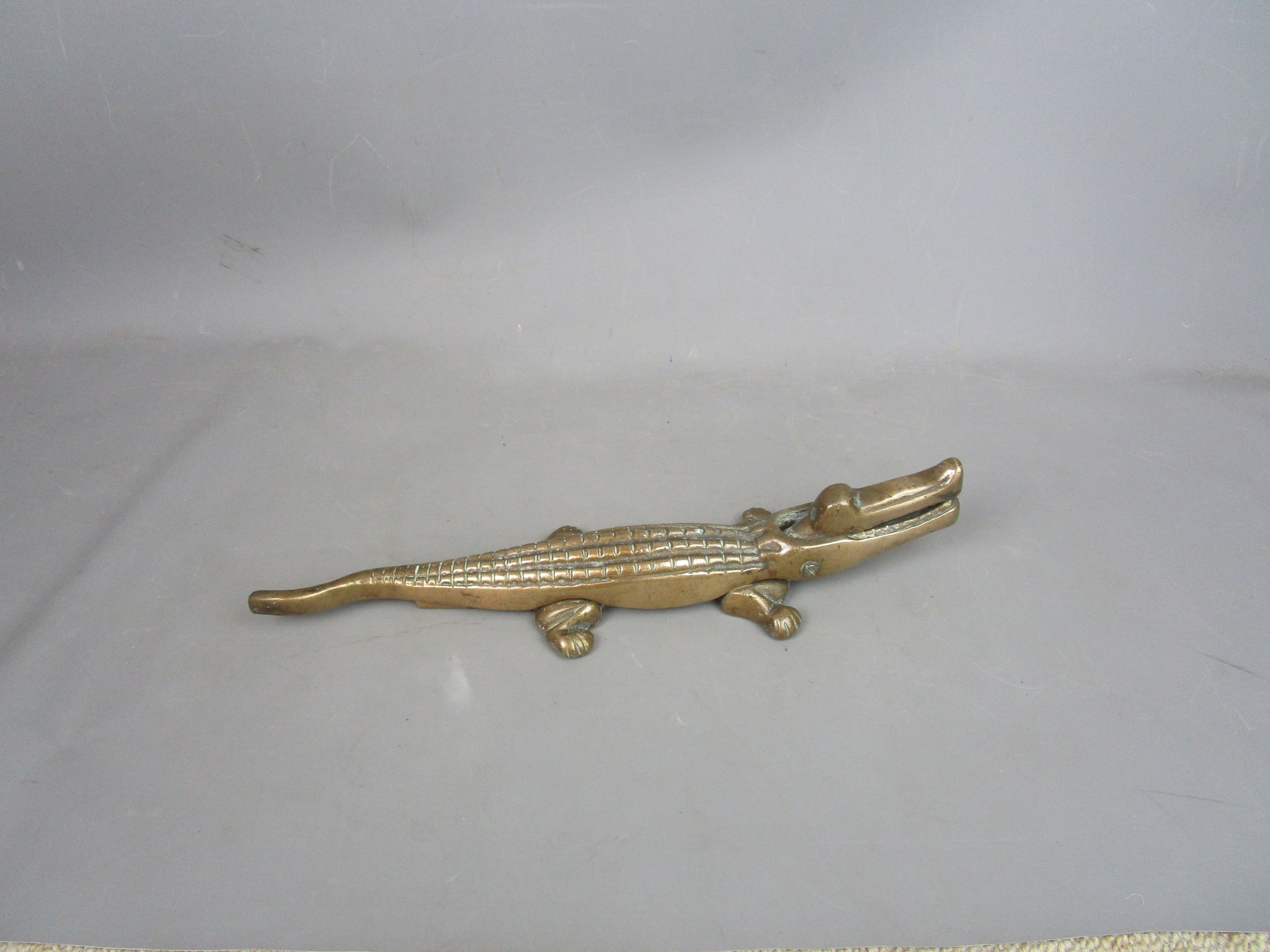This is a close-up photograph of a small, golden alligator statue approximately six to seven inches long, set on a surface that appears to be part of a bathroom or tabletop setup. The statue has a shiny, metallic finish with intricate grooves etched along its back to mimic scales, while the face, legs, and tail are smooth. The golden hue of the alligator is complemented by a hint of oxidized greenish color, adding depth and character to its appearance. The alligator’s body is positioned slightly below the center of the image, facing the top-right, with its tail extending towards the left. The face of the statue has a slightly open mouth, revealing a hint of detail around the eye and a small gap behind the head. The surface it rests on appears to be white, with part of a yellowish or white mat visible in the corner, peeking out from underneath a gray covering that folds up towards the back and has a noticeable crease. The overall setting is minimalist, with the alligator as the primary focus against a plain background.